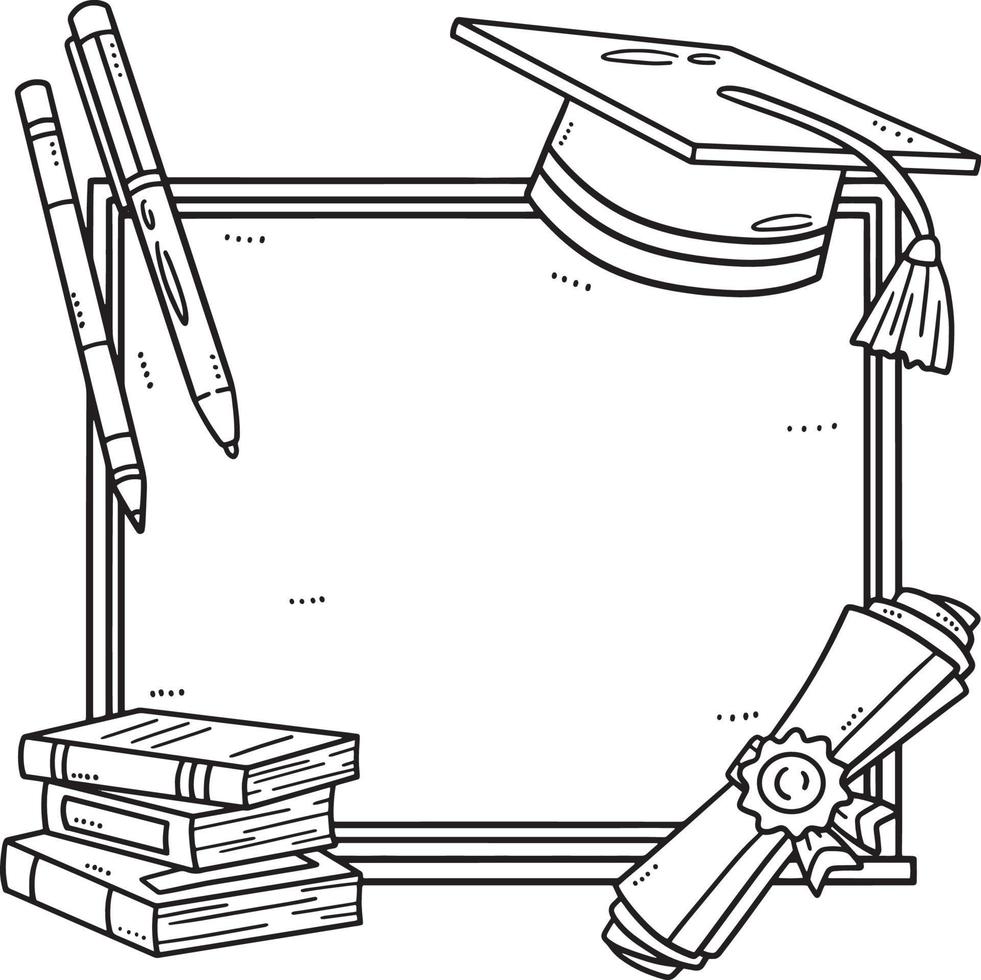This black and white drawing features a white background with a prominent rectangular chalkboard outline at its center, bordered by concentric squares. On the upper right corner of the chalkboard, there's a detailed drawing of a graduation cap, its tassel extending to the right and featuring a stripe around its side. The upper left corner showcases two writing utensils—a pen with a clip and a pencil—pointing downward. In the lower left corner, there is a stack of three uneven, horizontally-aligned books, each with subtle line details. The lower right corner depicts a rolled-up diploma secured with a ribbon. The drawing captures various academic elements, arranged meticulously around the chalkboard to create a cohesive and purposeful scene.